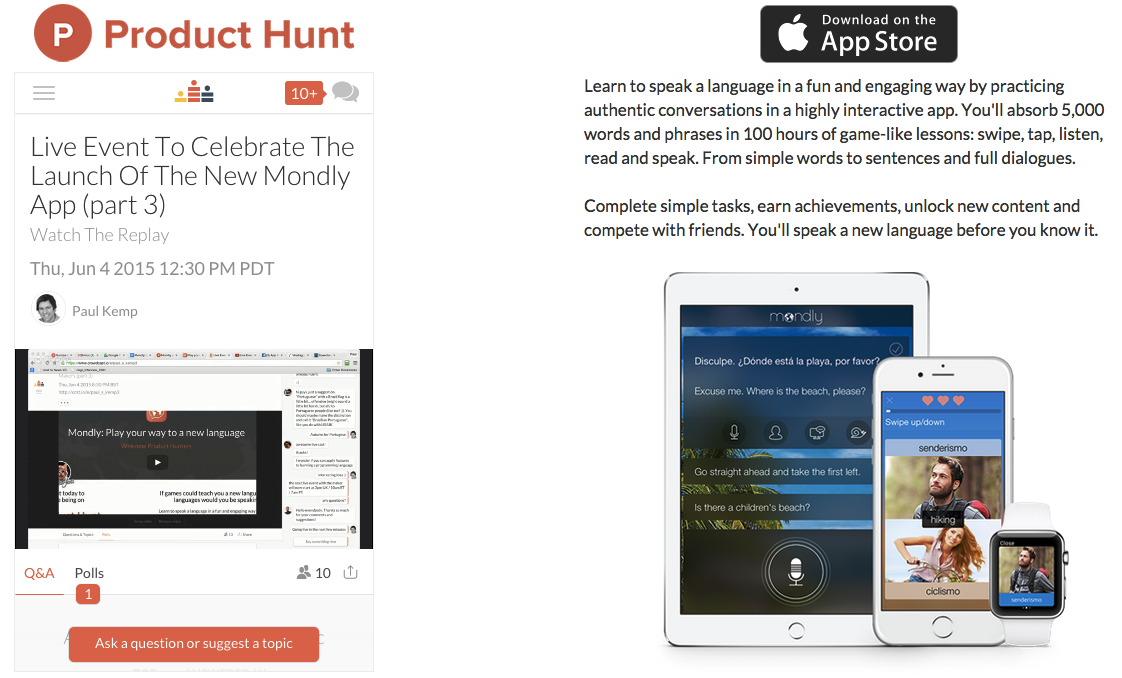The image is divided into two sections, with a screenshot on the left and another on the right. At the top, it features the text "Product Hunt" followed by "Live Event" to announce the launch of the new Mondili app, Part 3. The date and time of the event are displayed prominently at the top. On the left side of the image, details of the event are provided, while the right side includes a "Download on the App Store" button.

The caption for the image reads: "Learn to speak a language in a fun and engaging way by practicing authentic conversations in a highly interactive app. You can absorb 5,000 words and phrases in 100 hours of game-like lessons. Swipe, tap, listen, read, and speak, progressing from simple words to full sentences and dialogues. Complete tasks, earn achievements, unlock new content, and compete with friends. Speak a new language before you know it."